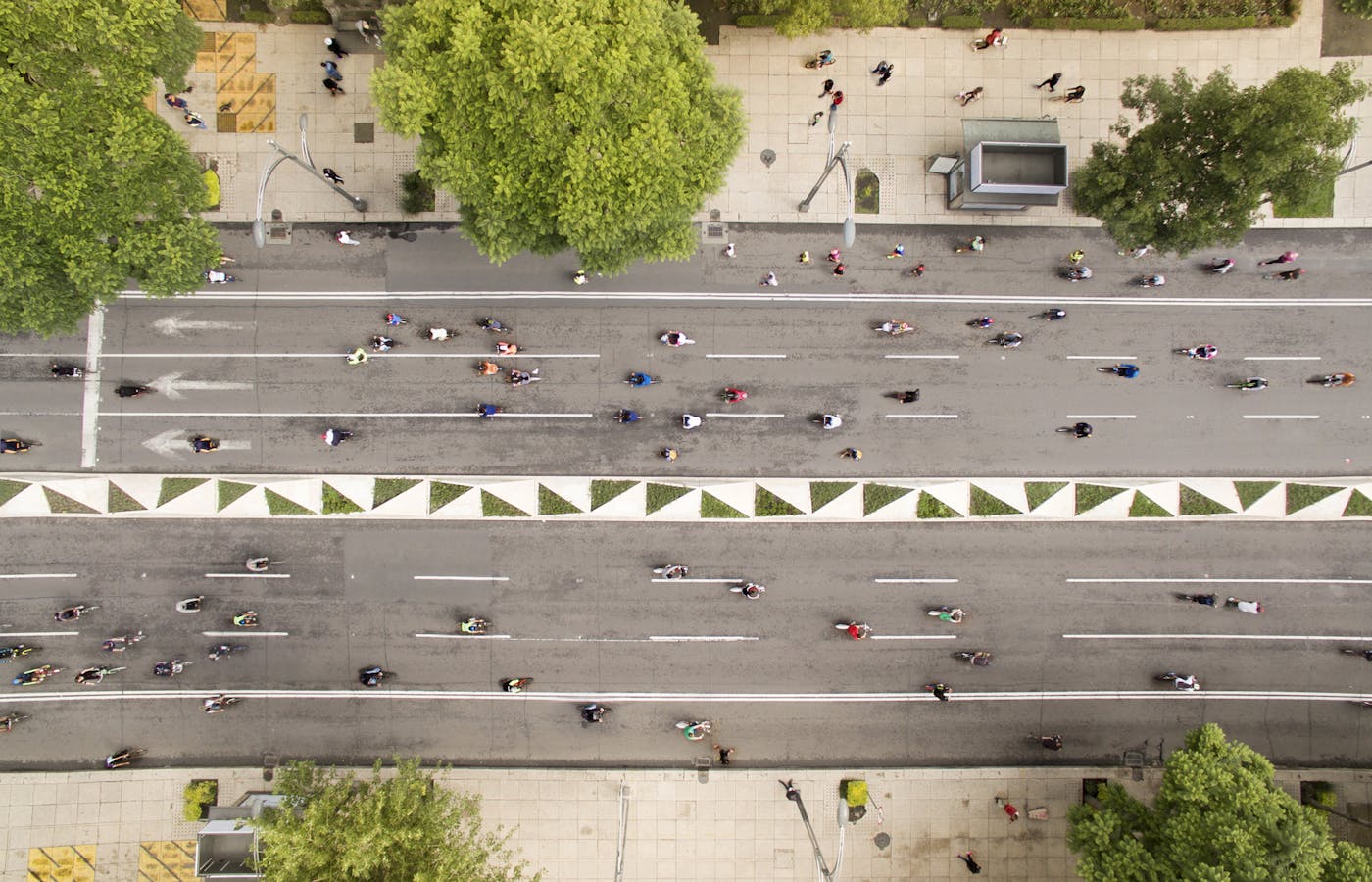An aerial view captures a bustling urban scene, centered on a gray two-lane road flanked by wide sidewalks. The road is divided by a narrow white median sporadically punctuated with small, green triangular islands. White lane markings provide orderly separation for the diverse, colorful array of cars navigating the roadway. The wide sidewalks, particularly prominent on the upper half of the image, teem with pedestrians in variously colored attire, indicating a vibrant city life. Streetlights and the tops of trees are visible, particularly where the bottom edge of the sidewalk is cut off from view. The scene suggests a typical day in a busy city, with residents possibly heading to work or other destinations.